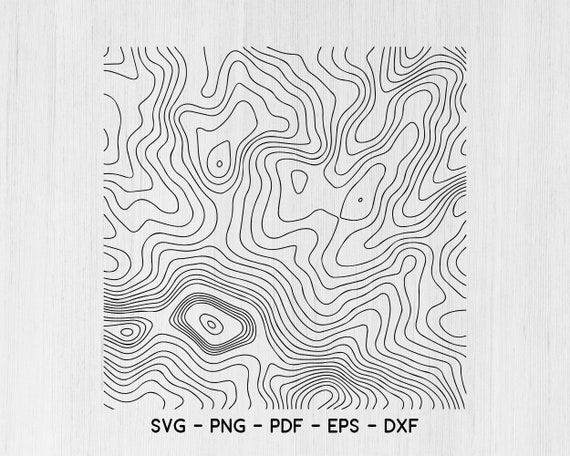The image is a squarish depiction set against a light gray, white wood-like background with darker vertical streaks. In the center, it features a complex black and white arrangement of squiggly lines and circles that resemble a topographical or radar map, or possibly even a set of fingerprints. The black lines intricately weave up and down through the white space within the squiggles, creating a detailed and abstract pattern. Among these lines, one prominent circle is encircled by several smaller dark circles. Beneath this central graphic, a series of file format designations are listed in capital letters: SVG - PNG - PDF - EPS - DXF. This text is distinctly placed at the bottom of the image, suggesting these may be the available formats for the graphic.